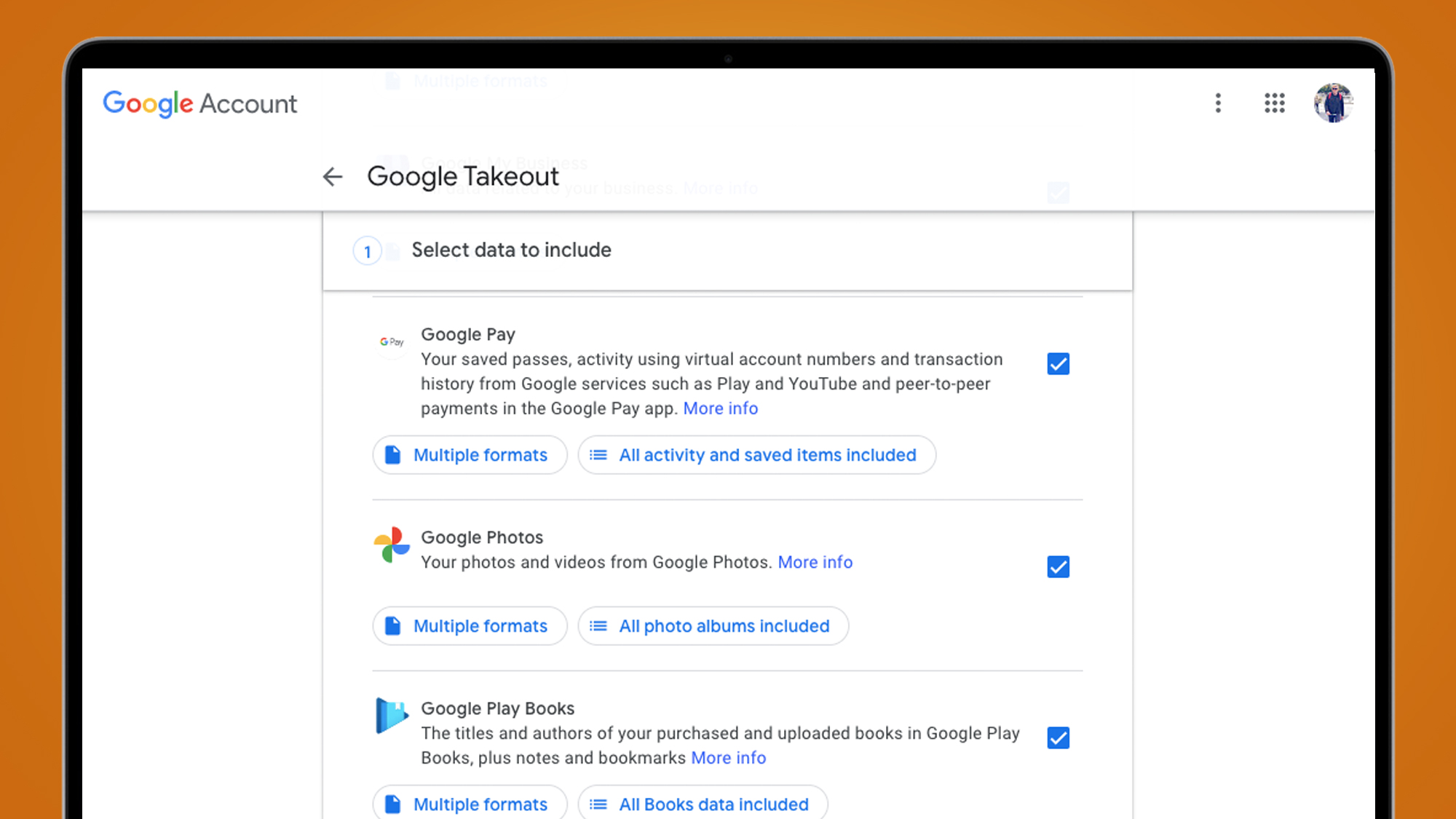The image features a detailed interface for Google Takeout, designed to help users download data from their Google services. 

The outer area of the image is shaded in dark orange, which transitions to black as it moves inward, creating a bold frame. In the top left corner, the words "Google Account" are displayed.

Moving down and slightly to the right, an arrow pointing left is placed next to the label "Google Takeout." Below, there is a numbered list starting with #1 indicating "Select data to include."

The first box covers Google Pay, described as "Your saved passes, activity using virtual account numbers, and transaction history from Google services such as Play, YouTube, and peer-to-peer payments in the Google Pay app." A blue box with a white check mark confirms that data from Google Pay is selected. Below this, users have the option to click on "Multiple formats" (highlighted in blue) and include "All activity and saved items" (also in blue).

The next subcategory is Google Photos, represented by an icon—a circle segmented in red, blue, green, and yellow—to the left. It details "Your photos and videos from Google Photos," along with options to choose "Multiple formats" and include "All photo albums," both highlighted in blue.

Finally, there is a blue arrow pointing to the right next to "Google Play Books," detailing "The titles and authors of your purchased and uploaded books in Google Play Books, plus notes and bookmarks." There is an option to click "More info" below, accompanied by a blue box with a white check mark confirming the selection.

This comprehensive overview allows users to understand the various categories of their Google data available for export.